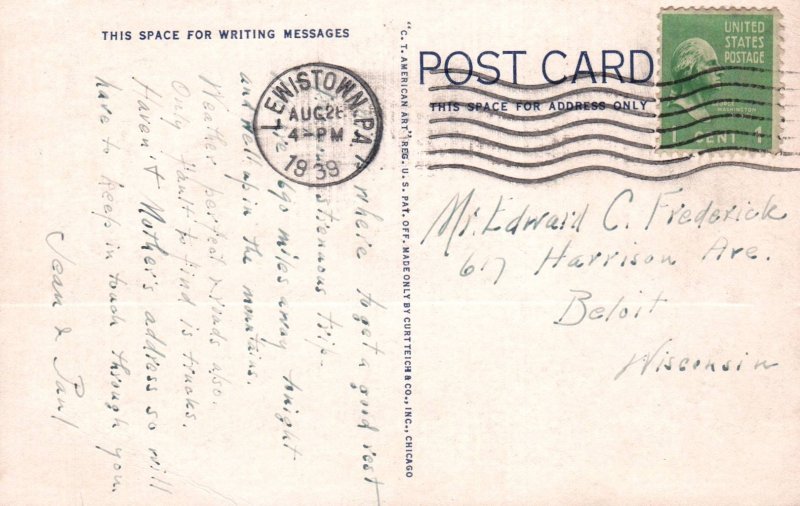This image depicts the back of a horizontally oriented postcard dating from August 26, 1939. The postcard measures approximately 5 to 6 inches in width and 3 to 4 inches in height. In the upper right-hand corner, there's a green 1-cent stamp featuring the portrait of President George Washington, with the white inscription "United States Postage." To the left of the stamp, in bold black letters, the word "POSTCARD" is printed, accompanied by the phrase "THIS SPACE FOR ADDRESS ONLY" and six wavy black lines beneath it. 

The postcard is addressed in black ink to Mr. Edwin C. Frederick at 617 Harrison Ave, Beloit, Wisconsin. Through the middle of the postcard, vertically, in black print, are the words "C.T. American Art Reg. U.S. Pat Off. Made only by Curt Teich & Company, Incorporated, Chicago." 

In the upper left section, there is a circular postal stamp from Lewistown, Pennsylvania, dated August 26, 4 PM, 1939. The upper part of the left side of the postcard, designated for writing messages, features a note in black ink that reads, "Haven't mother's address so we'll have to keep in touch through you," and is signed "Jean and Paul."